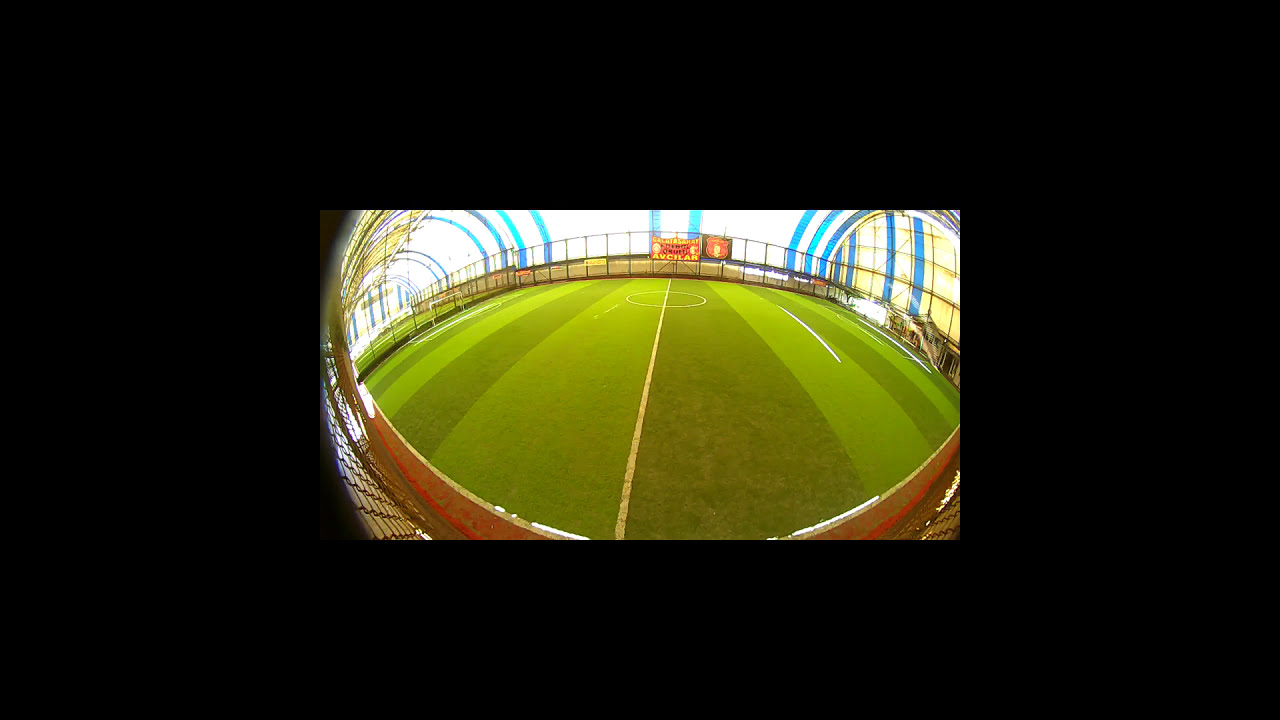The photograph showcases an expansive indoor soccer stadium taken with a wide-angle lens, lending the image a semi-curved, panoramic feel. The central feature is a meticulously maintained green soccer field adorned with alternating dark and light green vertical stripes. A distinct white line runs down the center of the pitch, culminating in a central circle. The field is framed by a brown and red-striped track, edged with silver and black fencing. The stadium's interior exudes a spacious, airy atmosphere, thanks to its glass walls and roof that slope upward. These glass panes are accented with bright turquoise and yellow striping, lending a dynamic, modern touch to the structure. The image is bordered by a thick black frame, emphasizing the brightly lit and colorful scene at the center. Notable details include white soccer goals at either end of the pitch, signs with partly legible text in yellow, red, and black near the top of the frame, and towering metallic structures supporting the roof. The walls feature striking white and blue stripes, contributing to the stadium's vibrant aesthetic. Overall, the scene is serene and devoid of players, highlighting the architecture and pristine condition of the field.